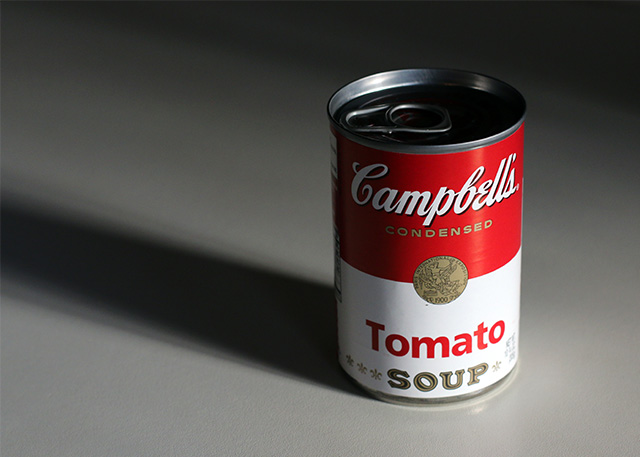The image features a stock photo of a Campbell's condensed tomato soup can. Set against a grey, textured table, the scene is brightly lit from the bottom right, casting pronounced shadows across the can. The metallic surface of the can reflects the intense lighting. The label is prominently visible, showcasing the classic Campbell's design. The top half of the label displays "Campbell's" in white text on a red background, followed by the word "condensed" in bronze. The lower half of the label is white, featuring a gold seal where the red and white sections meet. At the very bottom, the word "tomato" is printed in red font, with "soup" directly below in a blend of black and bronze fonts, adorned with additional decorative elements.